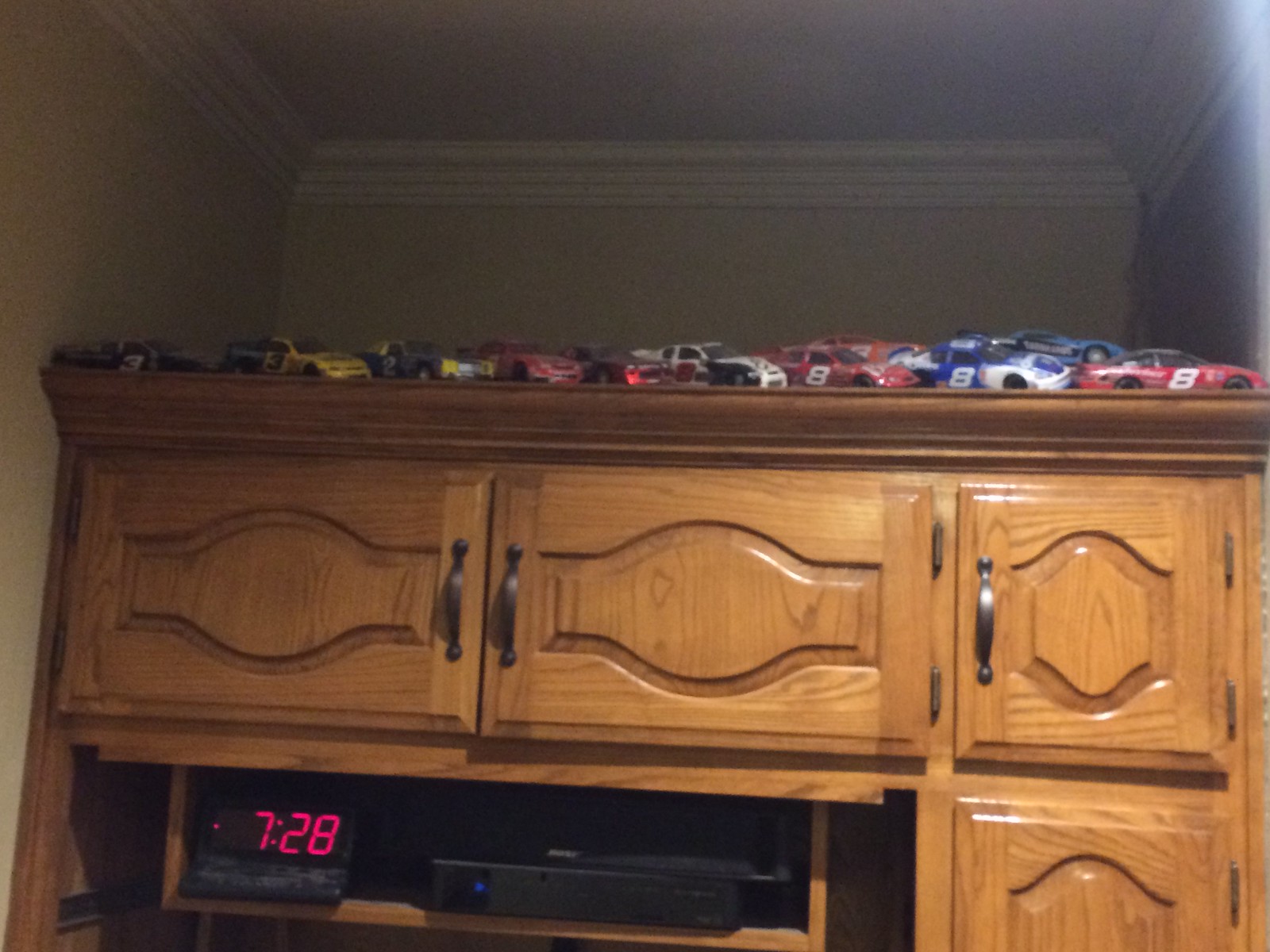The photograph depicts a section of a cream-painted alcove in someone's home, illuminated by a wall or overhead light. A wooden cabinet with decorative cupboards stands prominently within the alcove, topped with an assortment of colorful toy race cars. The collection features eleven cars, including several in black, red, white, and blue. Notably, three cars on the right display the number "8," while cars on the left bear the numbers "2" and "3". In the bottom left corner of the image, a digital alarm clock reading "7:28" is visible on a floating shelf, accompanied by what appears to be a satellite receiver box or radio modem. The ceiling and skirting are painted white, lending a clean contrast to the warm cream walls and the vibrant array of toy cars.